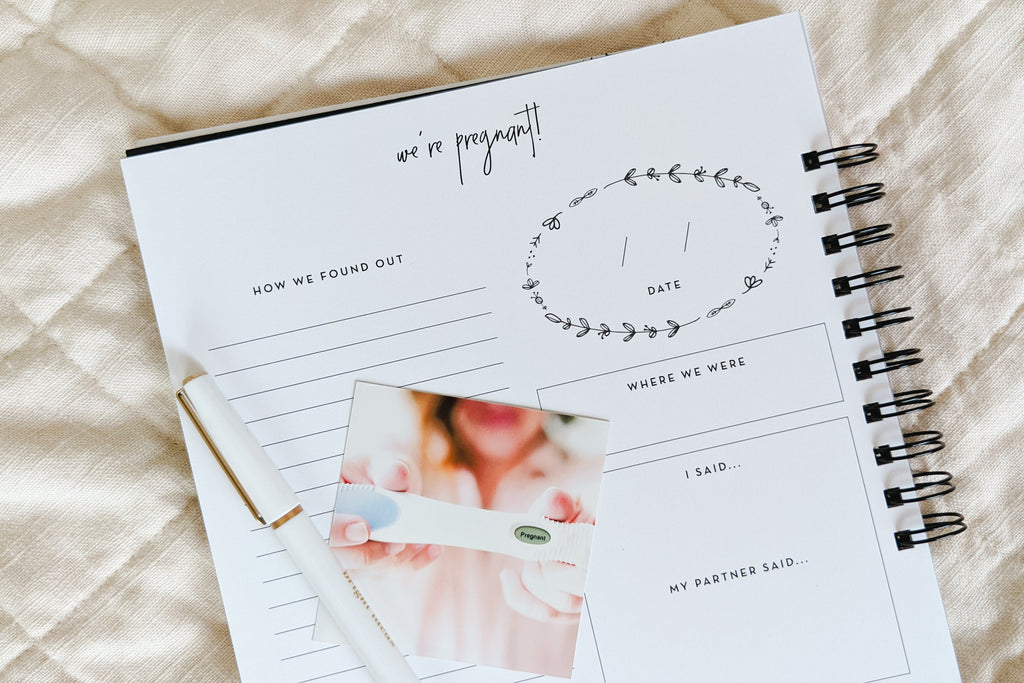The image showcases a detailed, brightly lit photograph of an open baby memory book resting on an ivory-colored blanket with visible stitching. The book is partially spiral-bound with black spirals on the right-hand side. The page open to view is designed to capture the moment of discovering a pregnancy, as it features several pre-printed prompts like "We're pregnant!" and sequentially follows with "How we found out," "Date," "Where we were," "I said...," and "My partner said...". Notably, there is a square photograph of someone holding a positive pregnancy test with the word "Pregnant" visible. Adding to the scene, a white pen with gold accents is placed on the page. The overall composition is clear, well-lit, and devoid of other distractions, highlighting the meaningful details of this special memory book.